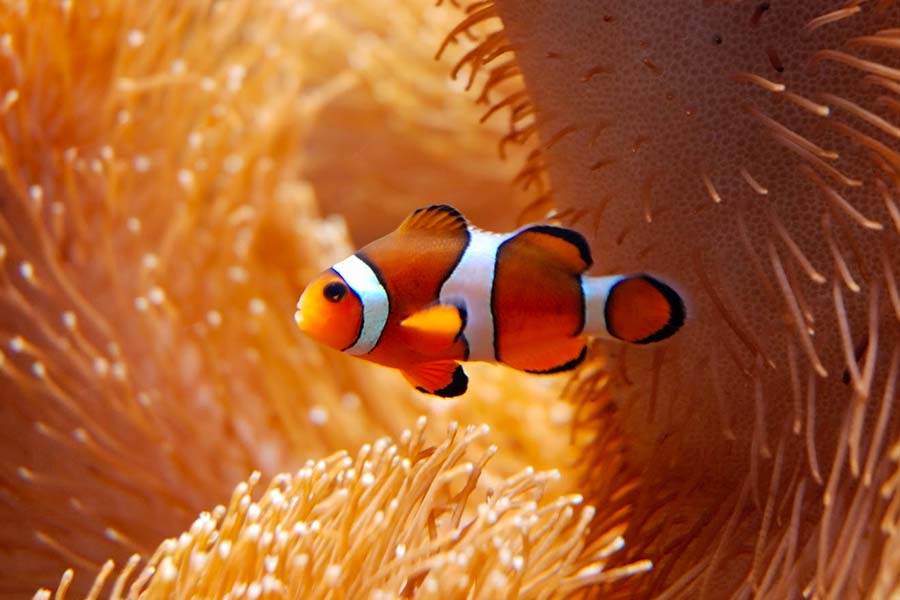This image features a vibrant clownfish, reminiscent of characters from "Finding Nemo." The fish is prominently positioned in the center, with its bright orange body segmented by three distinct white stripes—one behind its small black eye, one across its midsection, and one near the beginning of its tail. The orange hue of the fish varies in intensity, particularly vivid near the face and slightly darker towards the back. It has orange flippers and dorsal fins that appear to be in motion, giving the sensation of dynamic movement.

The background is densely populated with what appears to be a sea anemone, its sticky, tentacle-like structures showing a range of oranges from pale whitish-orange to deep, dark shades. This setting creates a captivating contrast and frames the clownfish beautifully, highlighting its striking coloration. The fish appears to be either suspended in animation or actively navigating its environment, adding a layer of intrigue and liveliness to the image.